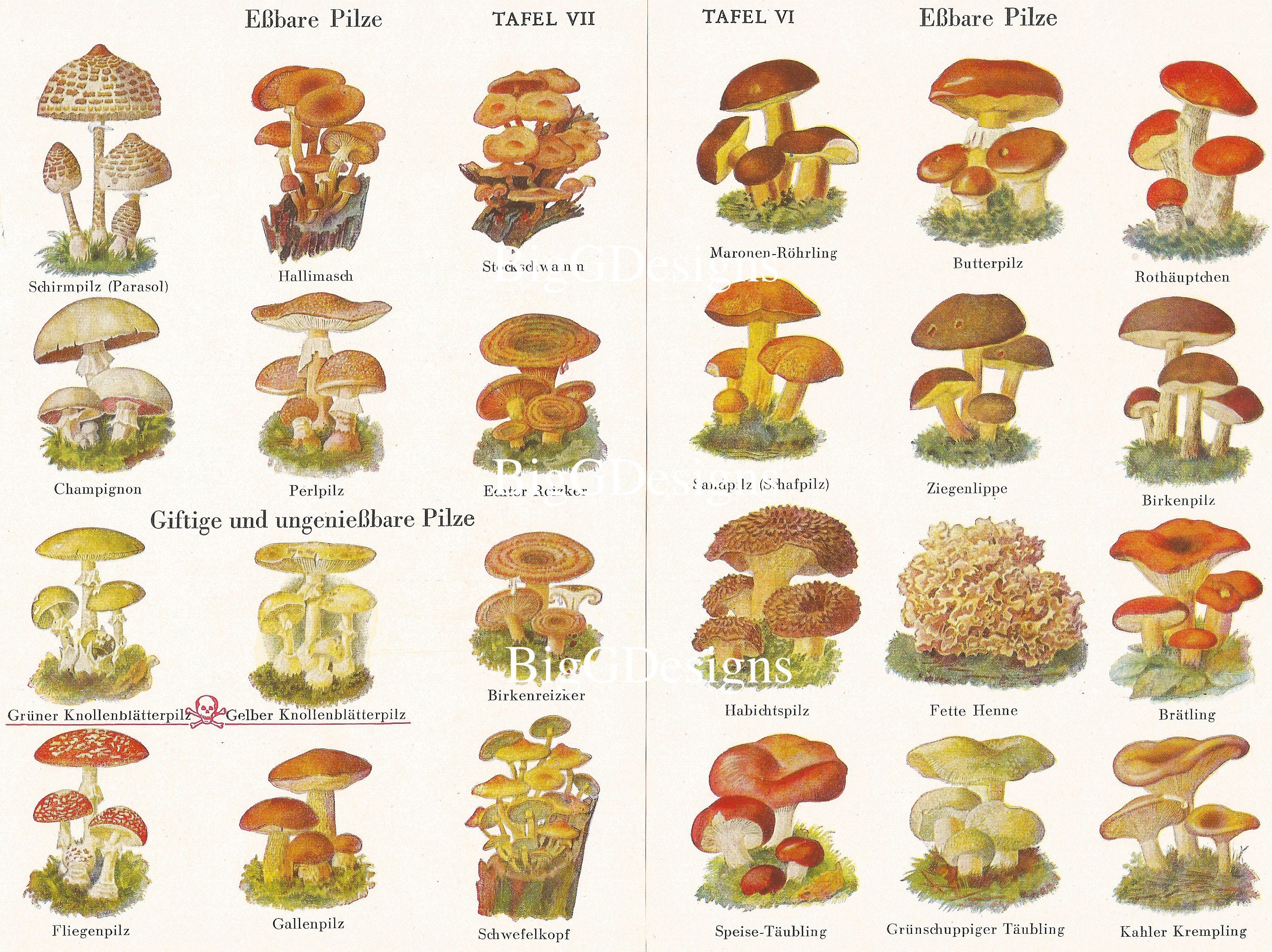This is a detailed hand-drawn illustration depicting 24 different varieties of mushrooms, appearing as a two-page spread from an opened book. Vibrant in its simplicity, each mushroom is meticulously labeled in a foreign language, indicative of an educational or botanical focus. The diagram showcases a broad spectrum of colors, including browns, yellows, oranges, reds, and even a coral-like shape, incorporating both common and unique species. Notably, one mushroom, named Butterplix, features a classic rounded red top. The layout consists of four rows and six columns, with each mushroom distinctly illustrated. Various texts throughout the illustration enhance its informative nature, and a watermark spans the book's spine, reading "Big It Designs," alongside a secondary watermark featuring a skull and crossbones.